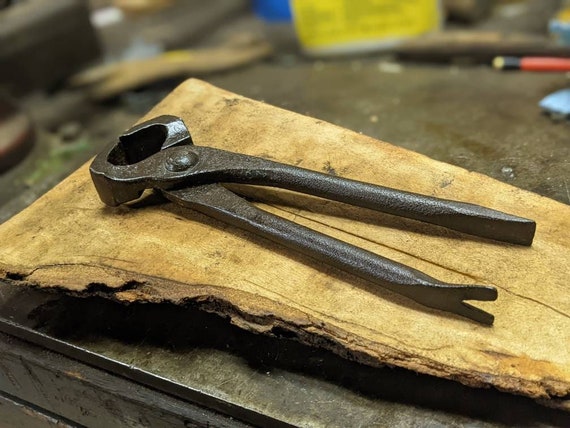This detailed photographic image, set indoors, captures an old, gray multipurpose tool, likely a special type of pliers with dual functions. One end of the pliers is wedge-shaped, possibly for chiseling, while the other end resembles a crowbar or hammer claw, suggesting it may be used for pulling nails. The pliers, currently closed, have a distinctive circular cutout near the top, giving them an oval appearance when viewed from above.

The tool is resting on a light brown, irregularly shaped piece of wood, prominently displaying its grain. The wood appears to be a smooth plank with a rough, bark-like edge, as though it's a freshly cut section turned upside down. This plank sits on a dark, aged workbench, which might be made of wood or metal, appearing grayish-brown with visible wear and tear.

In the blurred background, located in the upper right corner, are the tip of an orange pencil with a yellow eraser and a blue and yellow can or container, possibly glue, adding to the context of a well-used workshop. The visible details sharpen the focus on the foreground, where the worn tool and wood piece dominate the scene.